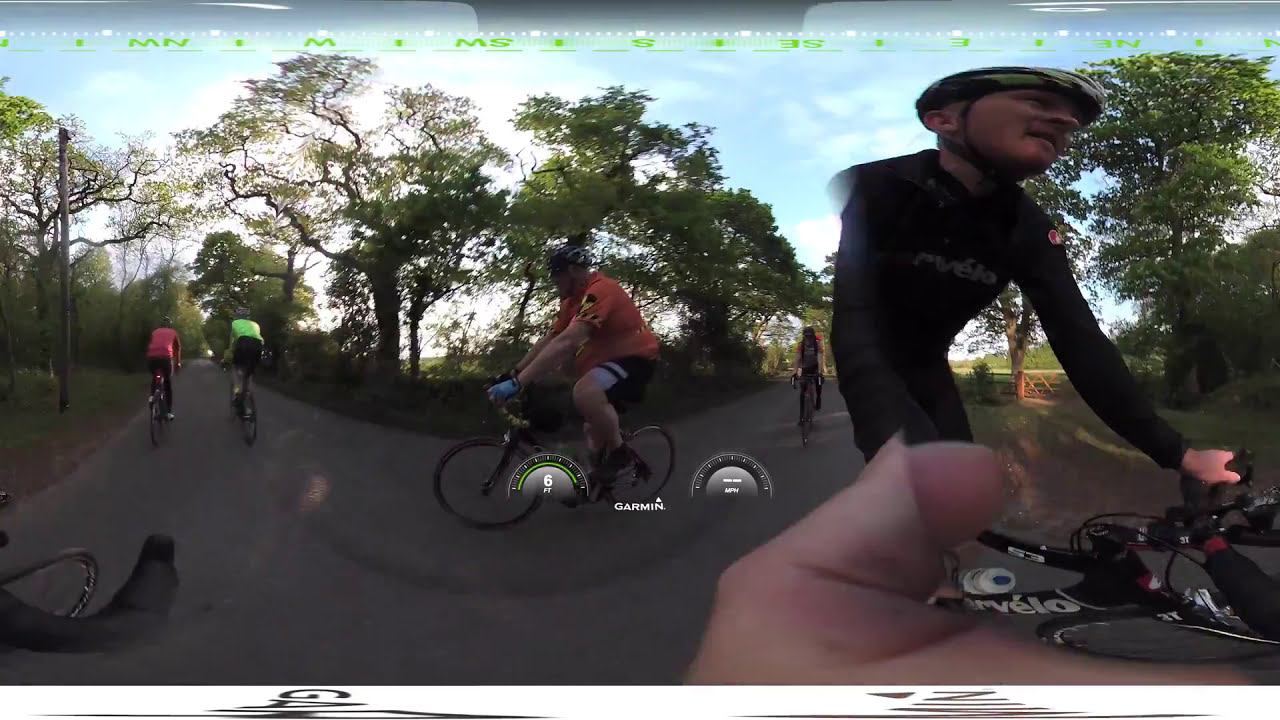The full-color, digitally enhanced photograph is an outdoor scene on a mostly sunny day with significant shadows covering most of the bike path. The rectangular image does not have a border. In the top portion, green text with M's, N's, and S's is added without obvious pattern. Several people are riding 10-speed bikes in different directions, indicating it's not a race. The central figure is an overweight man wearing an orange shirt and dark shorts, with the word "Garmin" and digital speed/distance readouts superimposed on him. The left side features another cyclist in a pink shirt, while a person in a green shirt rides further back. On the right, a cyclist in a tight black outfit and helmet, possibly the photographer, is seen with his thumb (covered by a band aid) distorting in the panoramic effect. The scene is shaded by trees with scattered sunlight illuminating a field in the background, blue skies, and some clouds. The image captures the angled handlebars, brakes, and controls of the bikes navigating the curved path amidst a lush, green environment.